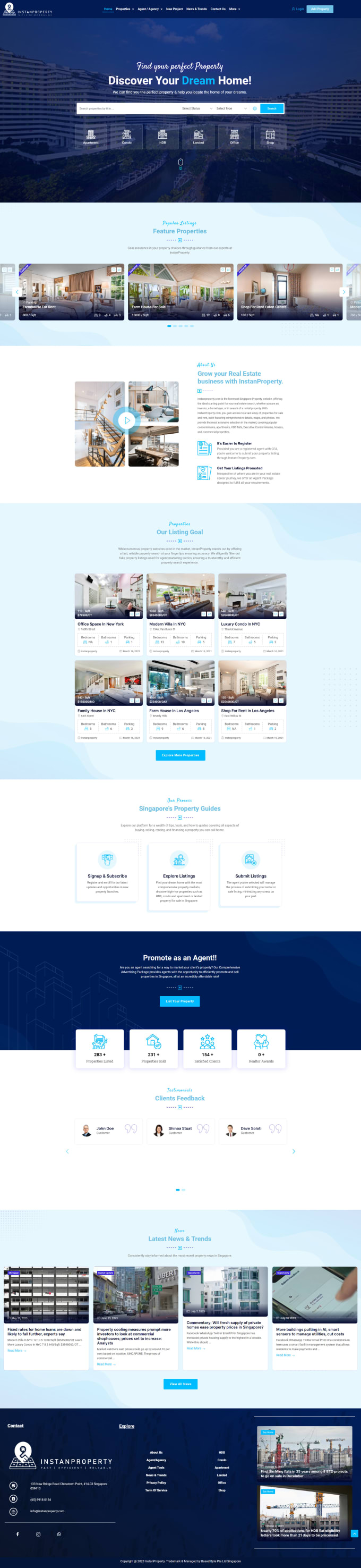A small, detailed screenshot of a double-page website layout. The top of both pages features a blue banner adorned with unidentified icons. Below the banner on the first page, there are three elongated photographs followed by two standard-sized photos and a block of text. Beneath this, two rows of three smaller, oblong images resembling interior photos are displayed. The second page mirrors this layout with a blue banner at the top, accompanied by four white tabs with blue text. Below, a white background hosts four elongated photos, each with accompanying text. The bottom of this page has another blue banner featuring a couple of pictures on the right side, with white text indicative of clickable links for further website navigation. The small size of the image makes it difficult to discern finer details.